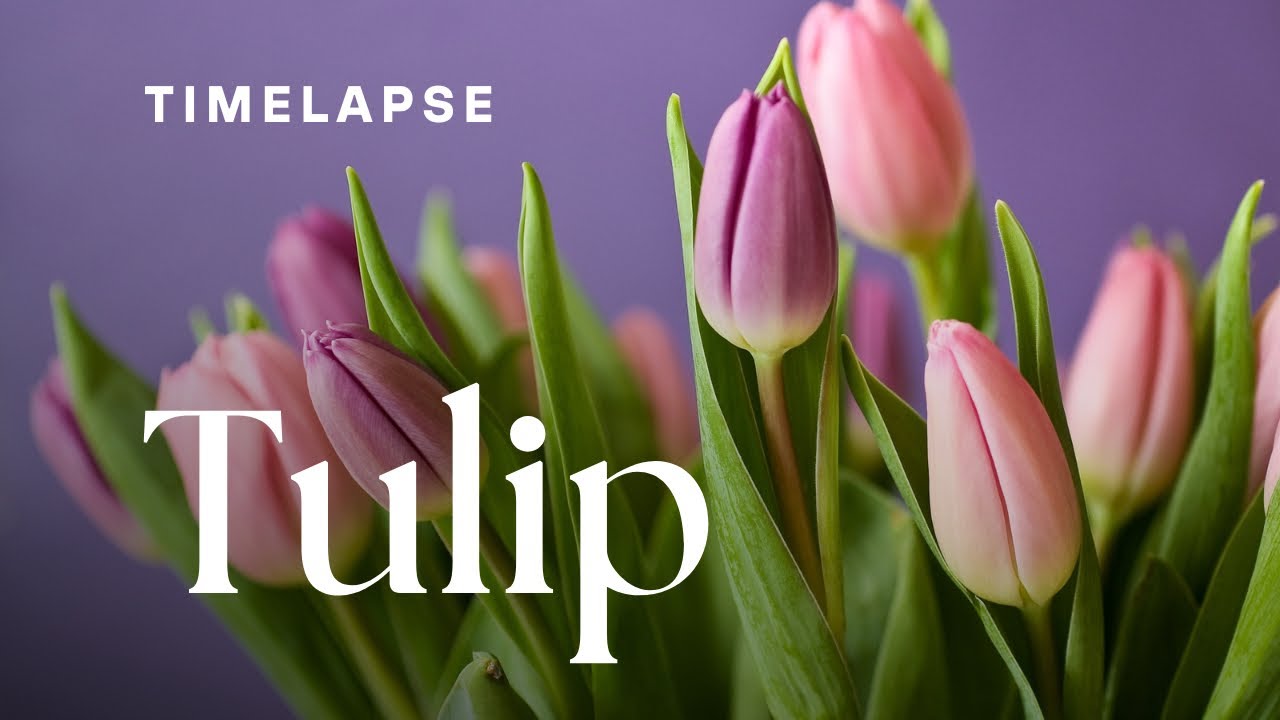This image features a vibrant and detailed close-up of a cluster of tulips that have yet to fully bloom. The pink and lavender petals of the tulips are still tightly closed, with their bright green leaves adding a lush contrast. The flowers stand prominently in the foreground, slightly centered and leaning more towards the right side of the image. The background is a deep purple, enhancing the colors of the tulips. In the upper left corner, the white all-caps text reads "TIME-LAPSE," and just below it, in slightly larger and bolder white text, is the word "Tulip." The image is in landscape orientation, capturing the delicate and unbloomed state of the tulips with a sharp focus on the flowers and a softer, more subdued background.